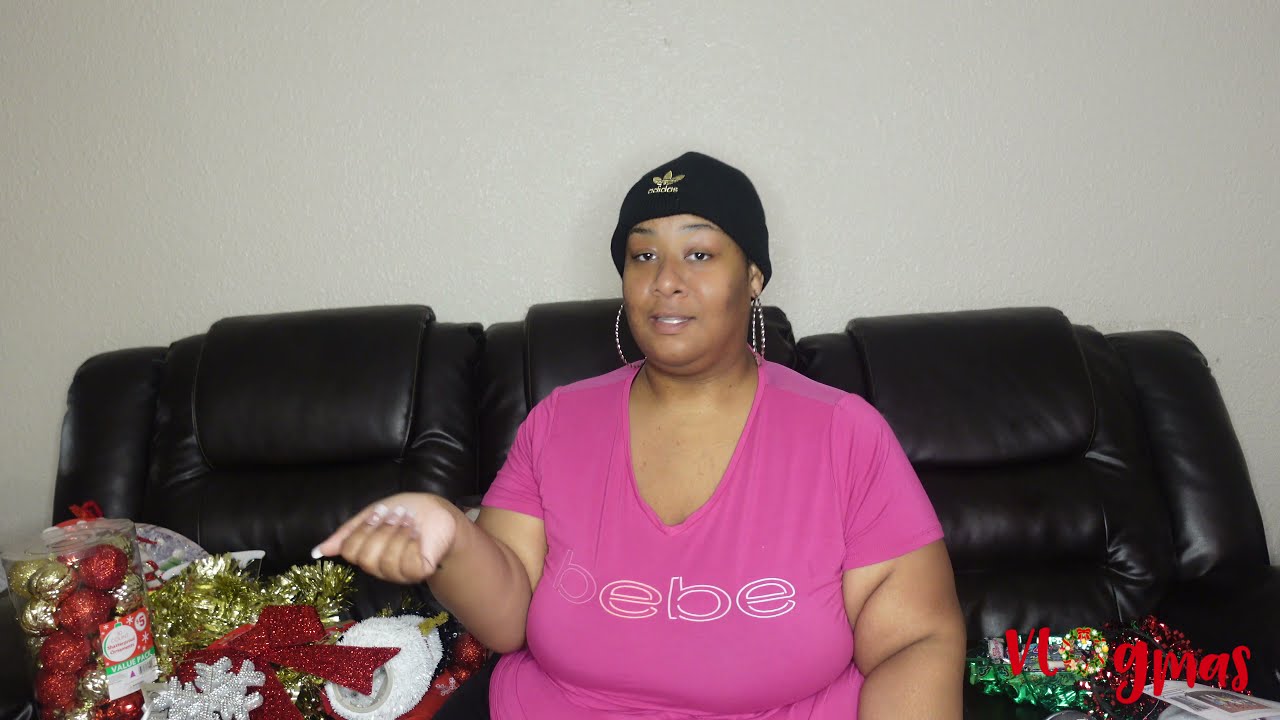In this color interior photograph, an African-American woman is seated on a glossy, black, three-piece leather couch, situated against a blank white wall. The woman, who is slightly heavyset, wears a black beanie with the Adidas logo emblazoned on the front and large hoop earrings. She dons a bright pink V-neck t-shirt that features the word “BEBE” spelled out as B-E-B-E across the front. Her right hand is held out in front of her, with her palm facing up and fingers closed, while her left arm rests at her side. She smiles softly at the camera, giving the image a positive and pleasant vibe. 

Around her, both to the left and right, are various Christmas decorations. These include red and gold garlands, shiny red and gold Christmas balls, and glittery red bows. Among the decorations, there are also stylized snowflakes and possibly Christmas lights. In the bottom corner of the image, there is text that reads "VLOGMAS," lending a festive holiday theme to the scene.